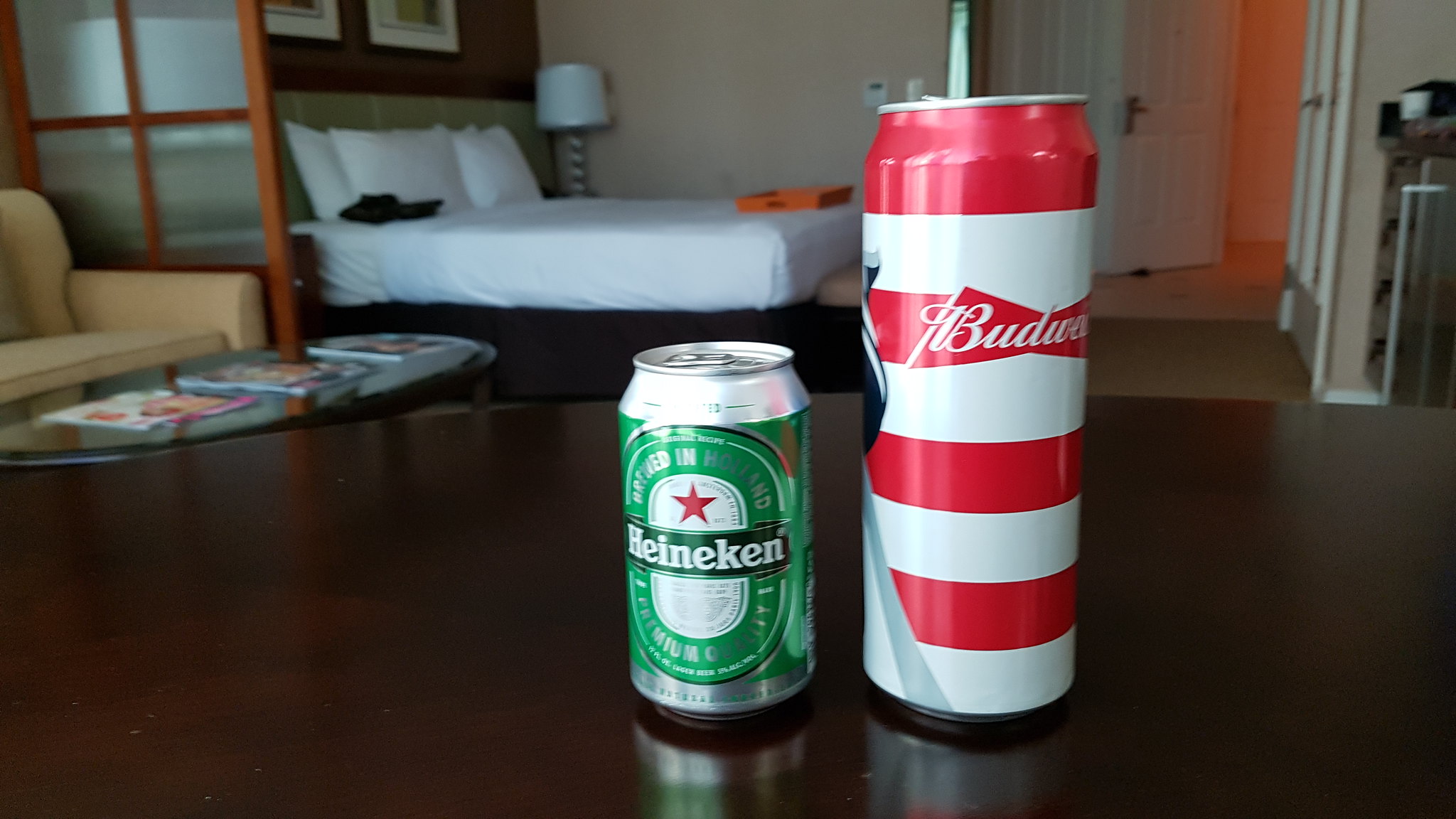This detailed colour photograph vividly captures two cans on a dark wooden table positioned centrally within a richly described room. On the left stands a standard-sized green and white Heineken can, prominently displaying the Heineken name across the middle in a green rectangle bordered by a green oval with silver text. A small white star is positioned above the logo. On the right, a significantly taller red and white striped Budweiser can, known as a Tall Boy, features a striking visual effect wherein the stripes at the bottom seem to peel off. The Budweiser logo nestles within a red bow tie shape emblazoned with white text on one of the stripes.

In the background, a beige couch or armchair and a coffee table stacked with magazines lend a cozy feel to the room. On the left, a wooden door with panels stands closed. A bed adorned with white sheets and pillows occupies part of the space, with a white or grey table leg lamp beside it. Above the bed, two pictures hang on a brown wall, contrasting with an adjacent grey wall. To the upper right corner, an open white door reveals another room bathed in orange light. A grey case or shelf with black objects on top sits near the door. The scene is completed with light brown flooring, adding warmth to the overall ambiance.